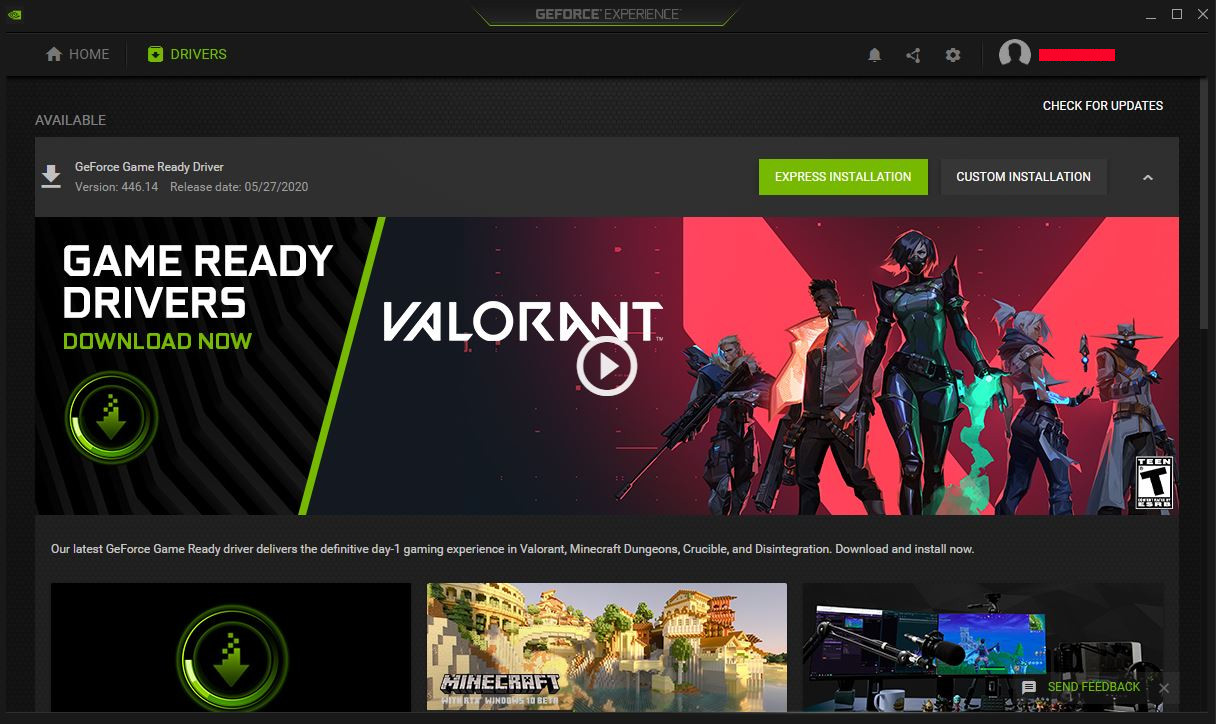Screenshot of the NVIDIA GeForce Experience application interface. The upper left-hand corner of the screen features a series of icons: a home screen icon in gray and a driver's icon in green, which is currently focused. On the upper right-hand corner, there are additional icons for notifications (a bell), settings, and the user's avatar.

Just below this, an "Available" label is displayed indicating that a new GeForce Game Ready driver is ready for installation. The name "GeForce" is stylized with a capital "G," lowercase "e," followed by capital and lowercase letters: "G," "e," "F," "o," "r," "c," "e." To the right of this label, two installation options are presented: a green button with white text that reads "Express Installation," and a dark gray button with white text that says "Custom Installation."

Underneath these options, there is a prominently displayed hero shot bar labeled "Game Ready Drivers - Download Now." Below this bar, a video thumbnail for the video game "Valorant" is prominently displayed. The thumbnail features several illustrated characters and includes a "Teen" rating icon in the lower right-hand corner.